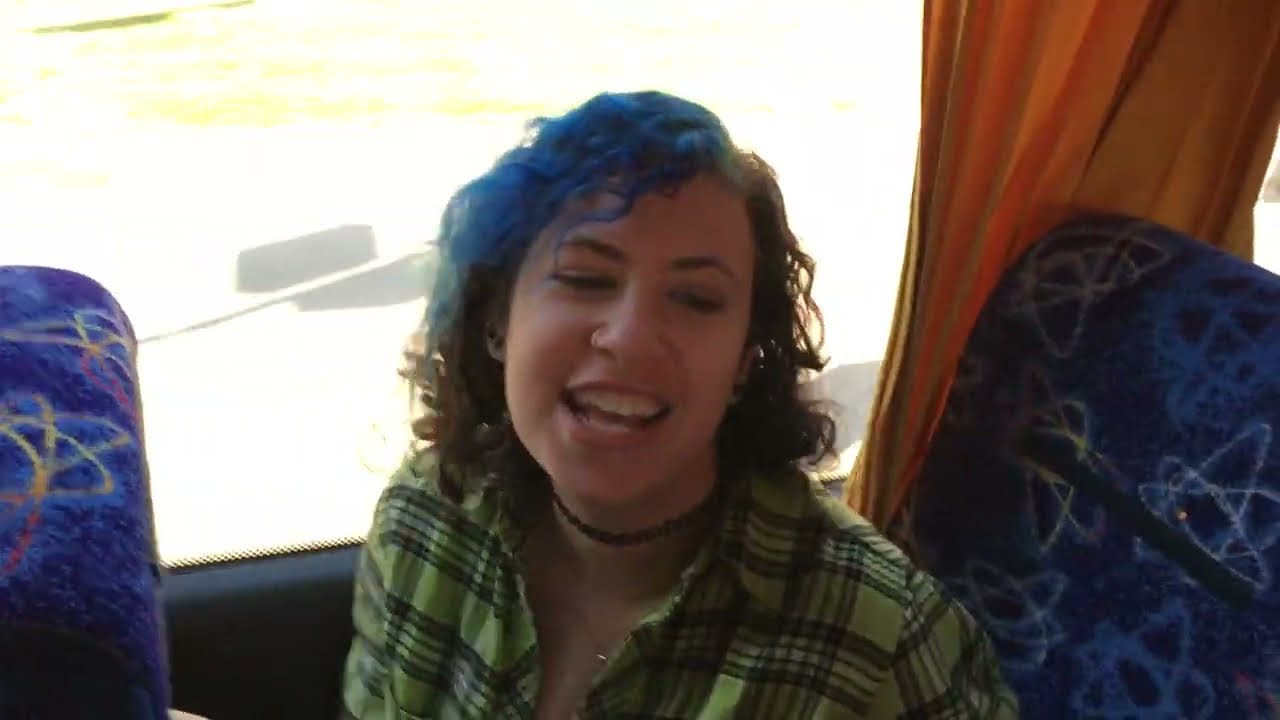The image shows the lively interior of a tour bus, brimming with animated conversation and youthful energy. The bus, potentially a coach or greyhound type, is filled to capacity with high school to college-age students. These young travelers are seated in uniform rows of two, their seats adorned with vibrant blue fabric featuring a Cosmos atomic design in various colors, including hints of purple and yellow. Most of the windows are draped in yellowish and orange curtains, likely tinted by sunlight.

At the forefront, a woman with distinctive half pink and half brown hair engages in a lively discussion or perhaps singing. Nearby, a teenager with light brown hair looks towards her with interest. The aisle is bustling; one girl stands with her phone, perhaps communicating with someone virtually. Many of the students are either standing or turned around in their seats, interacting excitedly with each other and particularly focused on one animated individual who appears to be the center of attention.

The atmosphere is jovial, with students wearing an eclectic mix of sunglasses, glasses, and hats, some leaning over seats to chat with friends. Despite the seemingly chaotic hustle, there's a palpable sense of camaraderie and shared excitement that fills the bus.